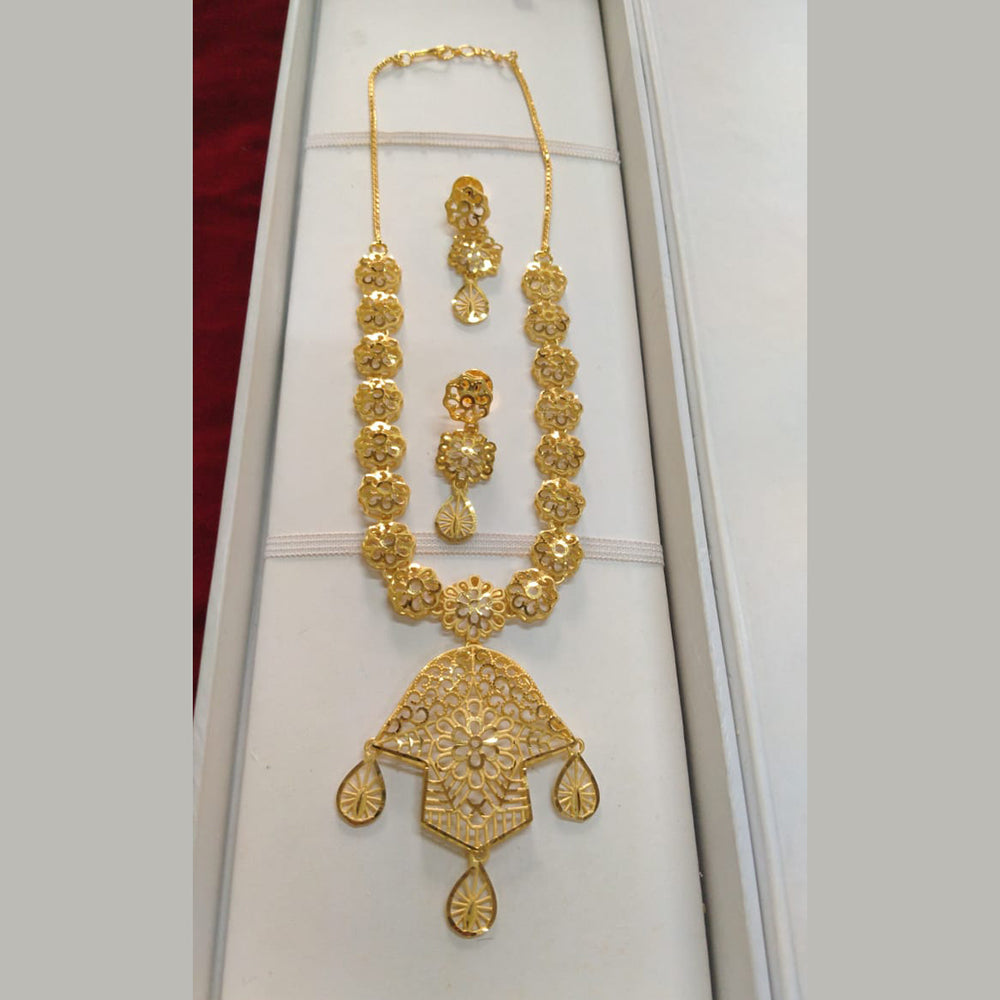This image showcases an ornate gold jewelry set elegantly displayed in a creamy white, vertically oriented box with a slight burgundy colored border on the back left corner. The background is white with a grayish border. The centerpiece is a traditional gold necklace featuring a herringbone chain at the back, secured with a small spring pull clasp. The necklace transitions into a series of about 16 intricate flower-shaped links, each resembling a flower with a central round element and petals, crafted in delicate filigree gold. The flower-shaped links create a beautiful U-shape design, culminating in a larger, more elaborate pendant with a mushroom cap shape, accented by three gold teardrop ornaments. Accompanying the necklace, and nestled in the middle of its loop, are two matching earrings, each mirroring the necklace's floral design with dangling teardrop-shaped pendants, all resting securely within the box's cushioned interior held by elastic straps.